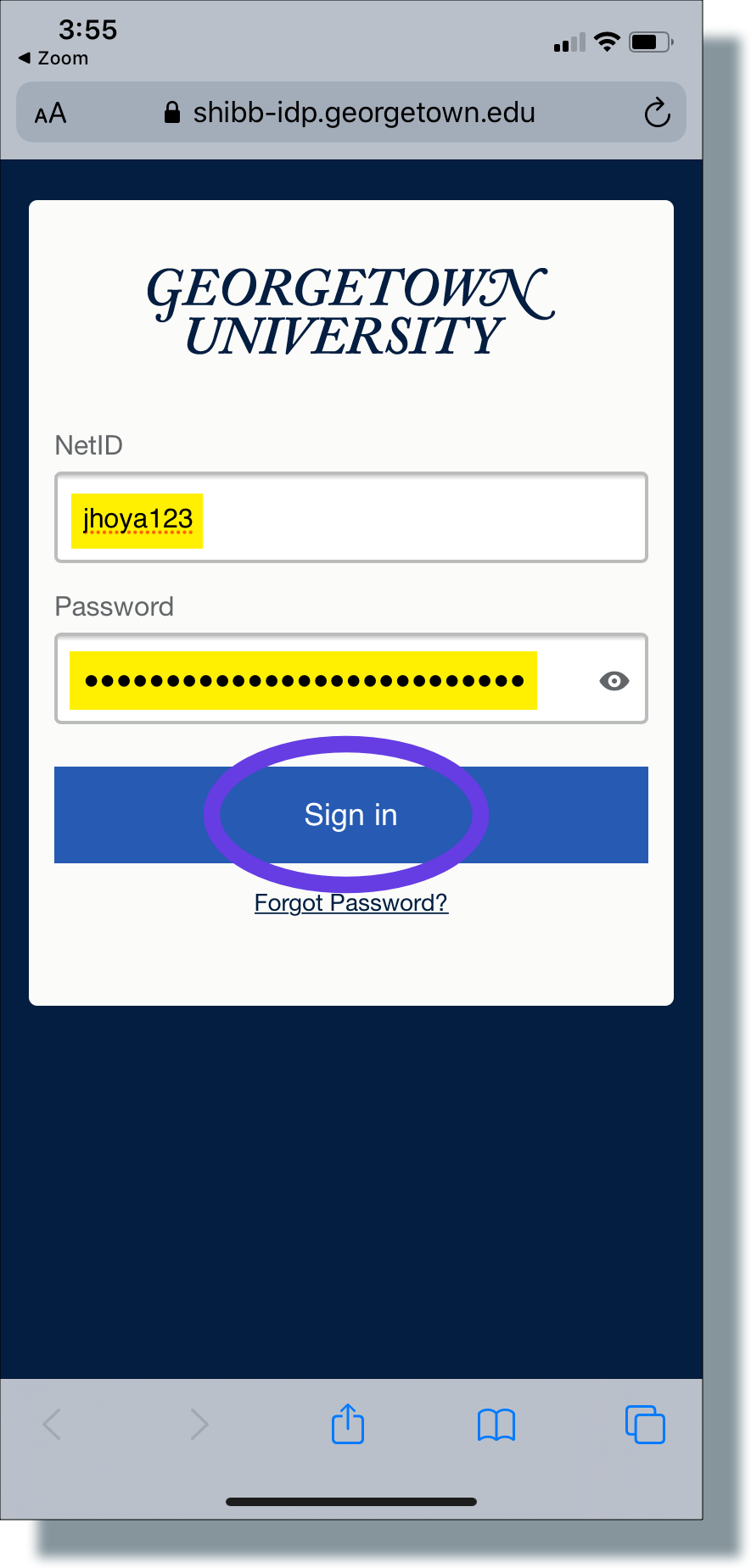This detailed caption describes a screenshot of a login page for a college website, specifically Georgetown University's portal. The image appears to have been captured from a smartphone, as indicated by the time displayed at the top left corner, which reads 3:55, and the battery icon at the top right corner, showing a bit over half full. The URL visible in the search bar at the top of the page is shib.idp.georgetown.edu.

The majority of the screen appears dimly lit, drawing focus to the brightly illuminated central section. At the top of this highlighted area, "Georgetown University" is written in italicized blue text. Below this, there are input fields for a NetID and password, each conspicuously highlighted in yellow. The NetID field contains the entry "JHOYA123," and although the password field’s content is obscured, it indicates a lengthy input, suggesting a strong password.

At the bottom of this central section, a prominent blue button with white "Sign In" text circled in purple is visible. Beneath this button, there is a "Forgot Password" link, providing users an option to reset their password if needed.